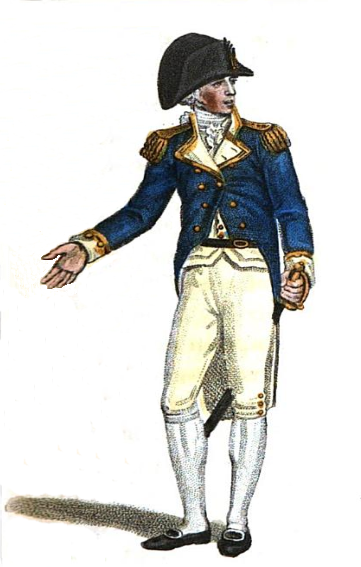This detailed drawing depicts a white military officer, resembling George Washington, dressed in Revolutionary War attire. He stands outdoors, his body casting a shadow to the left. The officer dons a tall, dome-shaped black hat tilted slightly to the left. His blue jacket, embellished with gold brass buttons and gold fringe on the epaulets and cuffs, is complemented by a ruffled white shirt with a gold-banded collar. A black belt cinches his waist, supporting a sword in its scabbard, which he holds with his left hand. His pants, terminating just below the knee, feature three buttons on the left leg. He is also wearing white socks and black loafers with either white or silver buckles. The officer's gaze is directed to the right and slightly upward, contributing to the commanding presence of the figure in the image. There is no text included in the drawing.